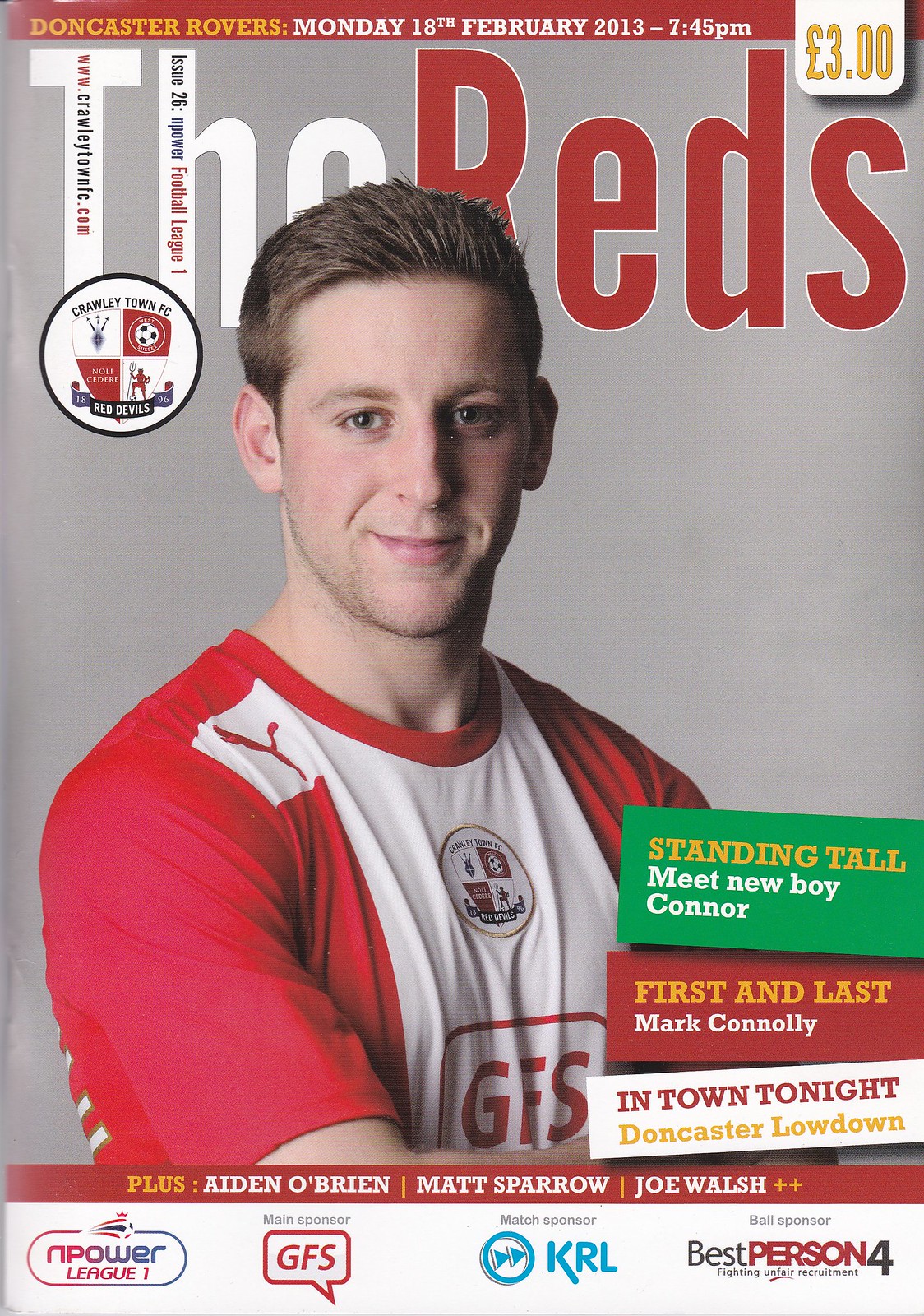This is the cover of the magazine "The Reds" featuring the Crawley Town Football Club, also known as the Red Devils. At the top, a red banner displays "Doncaster Rovers" in yellow, followed by the date and time "Monday, 18th February 2013, 7:45 PM" in white. The magazine price, "3.00 GBP", is noted alongside. The prominent central image is of a young white male soccer player, wearing a Puma jersey with red sleeves and a white torso, with the Puma logo in the middle of his chest. There’s a notable red circle with a soccer ball and four squares as part of the team's emblem. 

On the right side, three tabs convey key information against colored backgrounds: "Standing Tall. Meet new boy Connor," in white text on green, "First and Last," above "Mark Connelly" in yellow and white on red, and "In Town Tonight," followed by "Doncaster Lowdown" in red and yellow on white. The bottom section lists players Aiden O’Brien, Matt Sparrow, and Joe Walsh in white text on a red background, interspersed with small yellow plus symbols. Additionally, the sponsors, including Empower League One, GFS, KRL, and Best Person 4, are mentioned at the bottom of the cover.